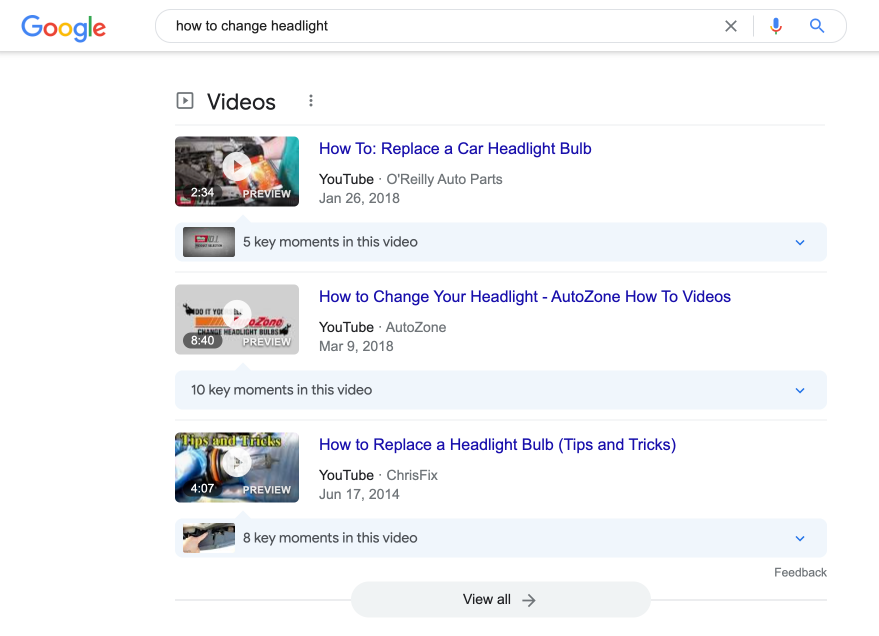This screenshot depicts Google search results for the query "how to change headlight." The page appears to be formatted for desktop viewing, with the Google icon prominently displayed in the upper left-hand corner, accompanied by the search bar containing the queried text in black font. Below the search bar, a thin grey line separates it from the search results.

The results section prominently highlights video tutorials. The top result, labeled "How to Replace a Car Headlight Bulb" in blue text, includes a small preview thumbnail on the left, which faintly shows an individual in a green shirt working inside a car. This video, sourced from YouTube, is from O'Reilly Auto Parts, dated January 26, 2018, and runs for 2 minutes and 54 seconds. Below the title, there is a blue band indicating "5 key moments" within the video, accompanied by a grey icon and a down arrow to its left.

The second result, titled "How to Change Your Headlight AutoZone How to Videos," also in blue text, features a preview image showcasing red, yellow, and black text on a grey background. This video, provided by AutoZone on YouTube, is dated March 9, 2018, and is 8 minutes and 40 seconds long. It has "10 key moments" indicated by a grey icon and a down arrow beneath the title.

The third and final video is labeled "How to Replace a Headlight Bulb: Tips and Tricks" in blue text and comes from the YouTube channel ChrisFix, dated June 17, 2014. The preview thumbnail features "Tips and Tricks" in yellow text at the top, with indistinct blue and grey elements visible behind a pointing finger. This video lasts for 4 minutes and 7 seconds and includes "8 key moments."

At the bottom of the screenshot, a grey rectangle centered with "View All" text and a right-pointing arrow is flanked by thin grey lines, suggesting additional video results can be viewed.